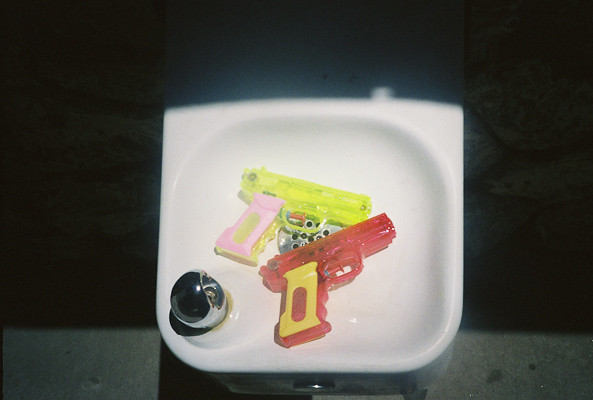The photograph showcases a white enamel drinking fountain, specifically a bubbler-type fountain, mounted on a dark, possibly black wall. The fountain features a stainless steel spigot and a silver button used to activate the water flow. The basin, which also includes a stainless steel drain, contains two small, translucent plastic squirt guns. One of the squirt guns is yellow with white handle accents, while the other one is reddish-pink with yellow handle accents. Both guns are inexpensive and their transparency reveals the interior where they would be filled with water. The background of the image is out of focus, highlighting a gray concrete sidewalk below the fountain.